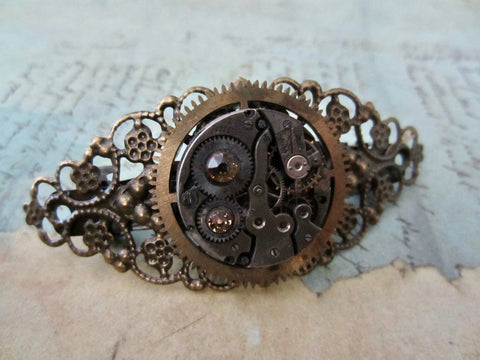The photograph showcases a detailed, steampunk-inspired piece of jewelry, likely a barrette or brooch, positioned in the center of the image. The item is constructed from a worn, coppery-brown metal and features intricate filigree designs. Central to the piece is a large, non-functional cog adorned with dark brown, topaz-like faceted stones, adding a decorative touch. Additional elements include smaller cogs, wheels, and bolts, alongside stylistic floral designs with five-petaled flowers at each end.

The background is a blend of two surfaces: a light blue, worn-out paper with cursive handwriting, possibly done with a fountain pen, and a beige marble or table surface. The blue paper, which appears to be torn or tattered, is overlaid on the beige surface, creating a layered effect. The cursive writing on the paper, written in a foreign language, adds a vintage aesthetic to the image, complementing the old-time charm of the steampunk jewelry. The overall composition accentuates the ornate and decorative nature of the central piece, making it appear as though it belongs in a steampunk costume or vintage collection.